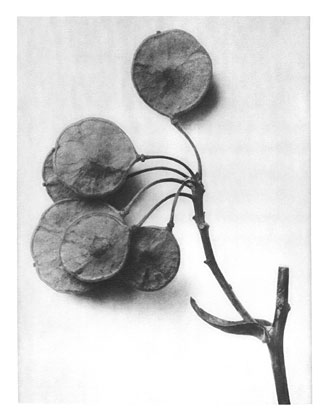This black and white image features what appears to be the dried seed pods of a money tree plant, artistically rendered in either charcoal, pencil, or captured through a high-contrast photograph. The composition is set against a textured off-white and gray background, which adds depth to the minimalistic piece. The plant's branch extends from the bottom right corner, giving way to round, coin-like seed pods. There are approximately five of these pods. One prominent pod sits unobstructed at the top, while others cluster to the left, connected by the central branch. The pods are characterized by their flat, circular shape with subtle shading in varying tones of gray and feature a slight bulge at the center, hinting at the seeds contained within. The overall aesthetic of the image is somber yet delicate, creating a distinct homage to nature. The piece lacks text, emphasizing its visual and interpretive simplicity.